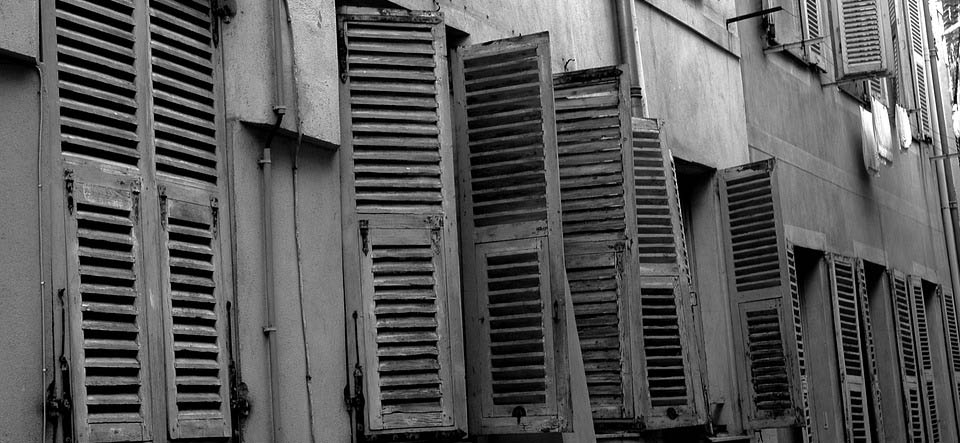This black and white photo captures the exterior of an old, weathered building, possibly composed of stone or concrete, characterized by numerous tall windows adorned with wooden shutters. The building appears to be an apartment complex. Some shutters, particularly those on the left and the far right, are closed, while others in the middle sections on both the first and second floors are partially open, providing a glimpse into the building's age and history. The image is taken from an angle, enhancing the visibility of the shutters' positions. Additionally, a metal pole runs vertically along the building to the right of the first set of shutters, accompanied by a cord that stretches along the right side of the pole. The overall weathered appearance of the shutters, coupled with their faded and whiter sections, suggests they have endured over time, contributing to the building's antiquated and storied ambiance.